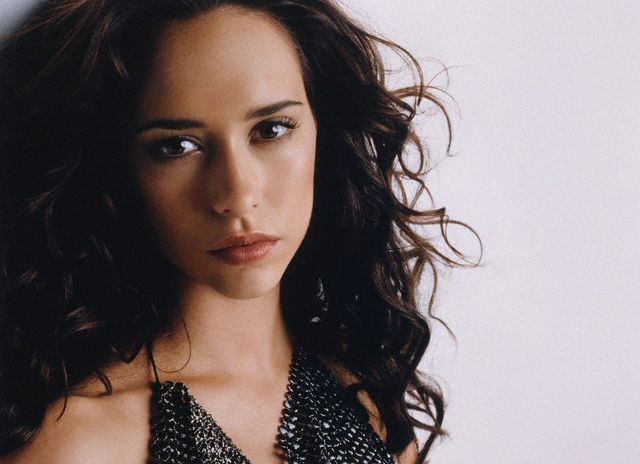In the photo, a woman gazes directly into the camera with a solemn expression. The frame captures her from just above the bust upward, showcasing her striking appearance. She wears a black, shiny sequin top that is elegantly secured with a single string around her neck. Her long, black hair cascades in full, wavy locks, complementing her darker skin tone. Her facial features are finely detailed: dark, well-defined eyebrows and deep, dark brown eyes framed by naturally long eyelashes. Her lips are well-shaped, and she has a delicate, small chin that harmonizes with her face’s overall contour. Her cheeks are subtly contoured, and her nose is proportionate to her refined face. Notably, she does not smile, adding to the intense and introspective mood of the image.